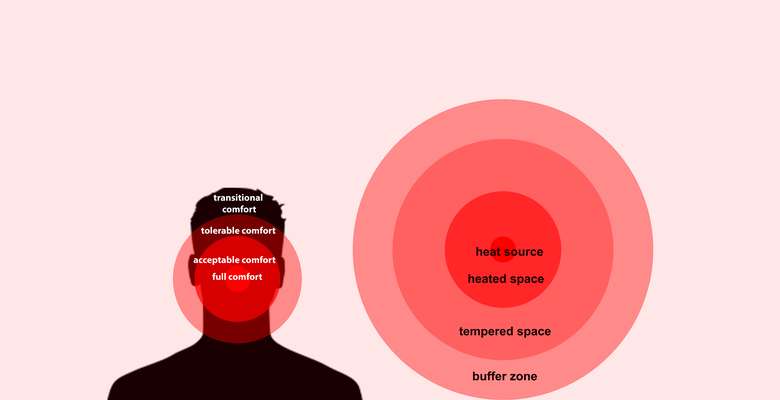The graphic image features a PowerPoint-style infographic set against a pale pink background. On the left-hand side, there is a black silhouette of a man's head and shoulders, with short hair. This silhouette is overlaid with concentric red circles of varying intensities that range from a dark red at the center to a lighter, almost pinkish red at the outermost ring. The circles represent different levels of comfort: the innermost circle labeled "full comfort", the next ring "acceptable comfort", followed by "tolerable comfort," and the outermost ring "transitional comfort."

On the right-hand side of the image, there is another set of four concentric circles also in varying shades of red. At the center is the darkest red labeled "heat source", the next ring is a lighter red labeled "heated space", followed by an even lighter red labeled "tempered space," and finally, the outermost pinkish-red ring labeled "buffer zone."

This detailed double-sided diagram illustrates the gradient of comfort levels around a head silhouette on the left and the gradient of heat zones on the right.